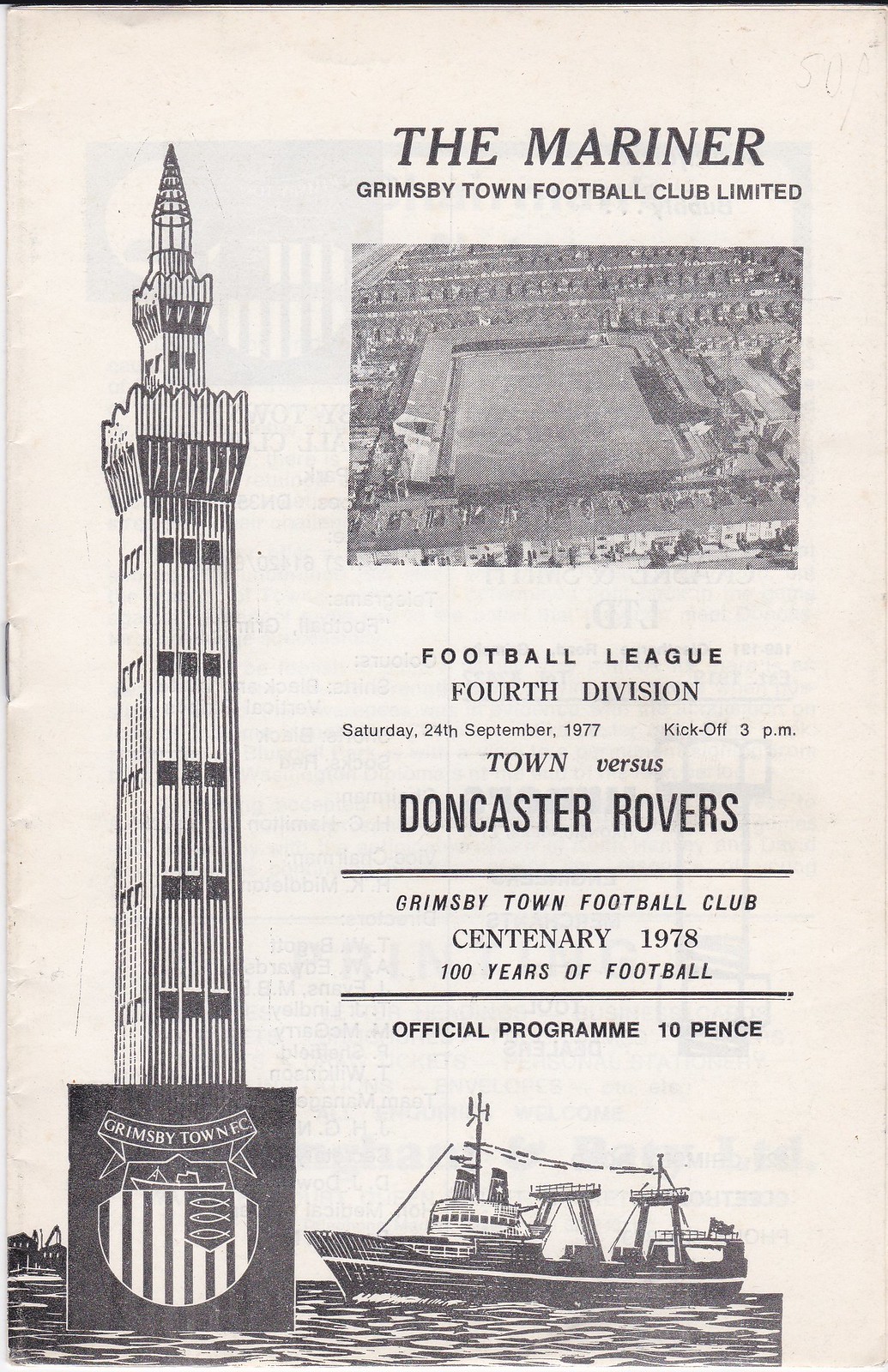The black and white cover of a football program from September 24th, 1977, prominently features the title "The Mariner: Grimsby Town Football Club Limited." At the center is a bird's-eye view photograph of the club's football field, where their 4th Division League match against Doncaster Rovers is scheduled to kick off at 3 p.m. Below this, text marks the club’s centenary celebration in 1978, highlighting "100 years of football." The official program, priced at 10 pence, also includes a vintage black and white image of a commercial boat sailing in a river. Accompanying this is the Grimsby Town NEC logo, designed as a shield with vertical stripes, depicting a boat, three fish, and a tall lighthouse with windows.